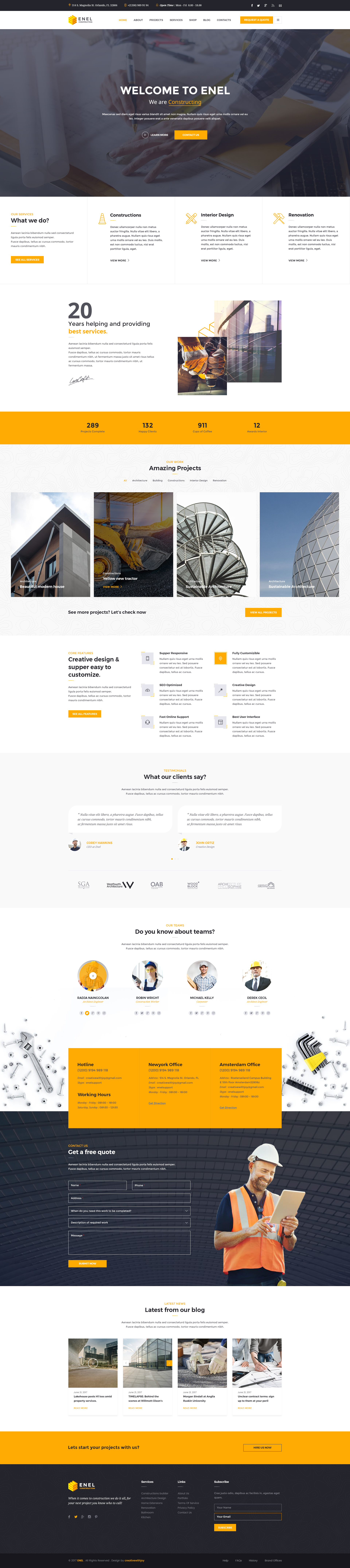This image is a screenshot of a website belonging to a company named ENEL. The layout appears stretched horizontally, making it challenging to decipher the text clearly. The site's banner reads, "Welcome to ENEL" and mentions their involvement in construction. The next visible section notes their 20 years of experience in the industry, highlighting their dedication to providing the best services in interior design and renovation.

Beneath this, the website displays some statistics that are partially obscured, including "289 checks completed," "132 happy clients," and "911 cups of coffee." Further down, there's a showcase of four project photographs followed by additional text content. The dominant colors of the website are black, orange, and white, with other accent colors like yellow, gray, and blue contributing to the overall design. Despite the distortion, the website presents ENEL's commitment to construction and design services through vivid imagery and structured content.